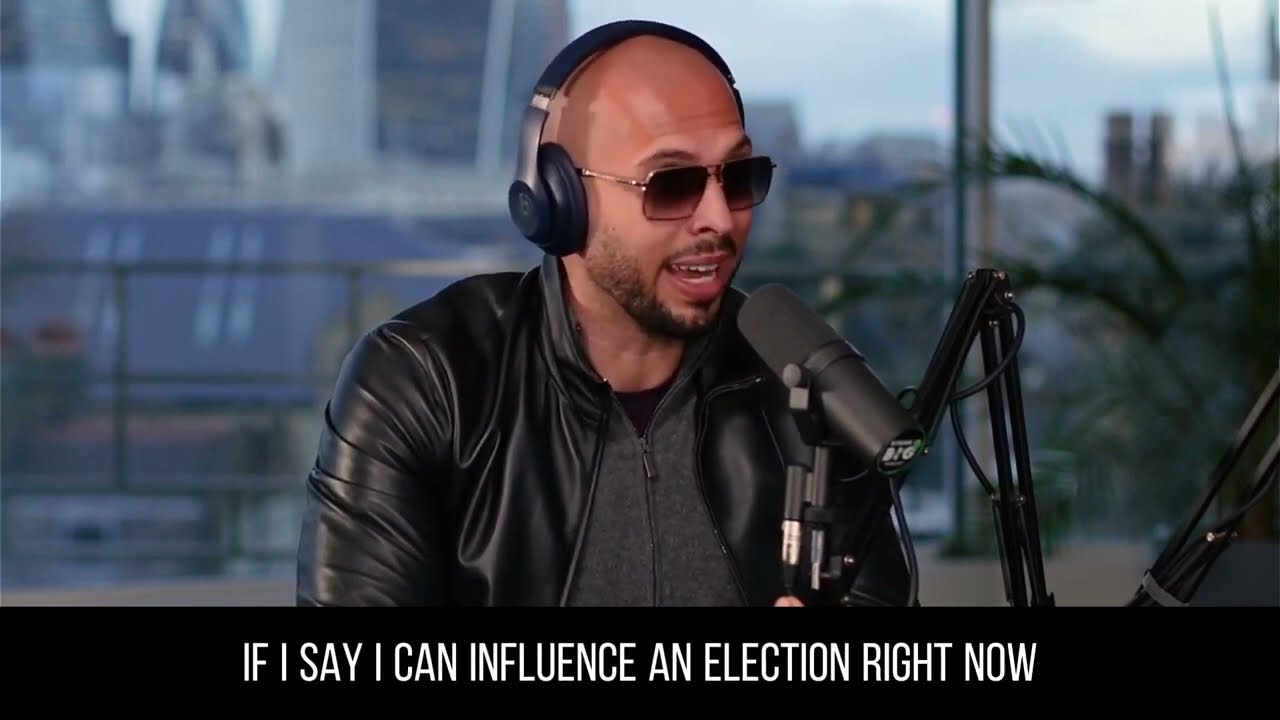The image captures a black man with very short hair and a balding front, wearing black sunglasses and over-the-ear headphones, speaking into a black microphone on a black stand. He sports a goatee with a thicker patch of hair on his chin and a thin mustache extending across his upper lip. The man is dressed in a black leather jacket, a dark gray zippered sweater, and a black t-shirt underneath. He appears to be happy, speaking mid-sentence with his mouth open, revealing both his top and bottom teeth. He is facing slightly to the right, at a diagonal to the viewer. The backdrop features a large window through which a large blue building with white roofs and two centered towers can be seen, along with the dark silhouette of a palm tree leaf. A black bar at the bottom of the image displays white all-caps captions that read, "IF I SAY I CAN INFLUENCE AN ELECTION RIGHT NOW." The entire background behind the man is slightly out of focus, emphasizing the indoor setting, possibly a studio, with a plant visible to the right.